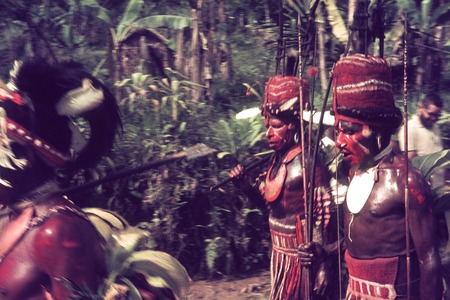In this vibrant and captivating image, we observe a group of indigenous tribal men standing in a lush, tropical jungle setting amidst greenery including banana leaves and palm trees. The three central figures, all dark-skinned, are adorned in traditional tribal attire. Their faces are strikingly painted with red and white markings, accompanied by dark paint around their eyes. Each man is bare-chested, wearing ornate white and red necklaces and distinctive red high headdresses. They also donn red pelt-like loincloths or high skirts around their waists. Additionally, these men appear to be holding primitive weapons, possibly spears or bows and arrows. On the far right side of the image, slightly in the background, a white man dressed in a casual white t-shirt, possibly a tourist, stands observing the scene. His presence contrasts sharply with the richly detailed traditional attire of the tribal men.